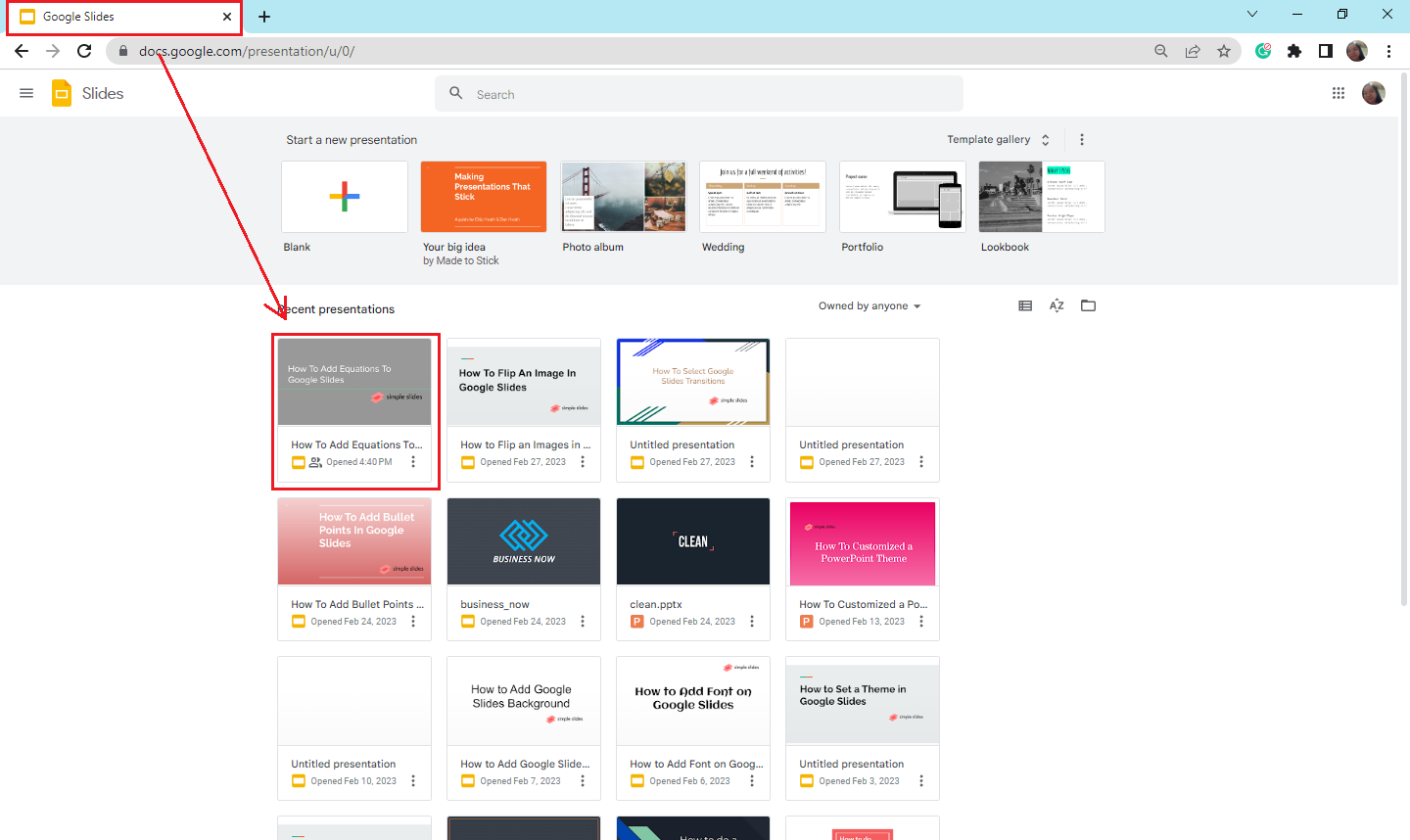The screen displays the Google Slides homepage from docs.google.com. A prominent red arrow directs attention diagonally downward from the "Google Slides" heading to a specific area below. Initially, below the main heading, there's a "Start a New Presentation" section offering six template options: Blank, Your Big Idea, Photo Album, Wedding, Portfolio, and Lookbook.

Further down, the "Recent Presentations" section showcases twelve presentation thumbnails arranged in a 4x3 grid. The red arrow points specifically to the first thumbnail in this "Recent Presentations" section. This highlighted thumbnail, labeled in bold gray text as "How to Add Solutions to Google Slides" from Simple Slides, indicates that the presentation covers guidance on adding solutions to Google Slides. Additionally, it notes that the presentation was last opened at 4:40 PM.